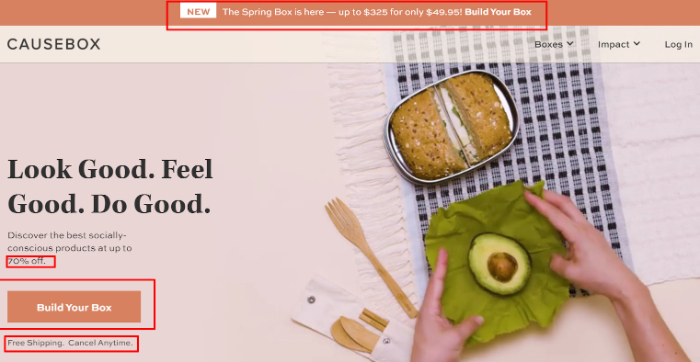The webpage for Causebox showcases an enticing layout with an orange navigation bar at the top. A prominent red box highlights the text proclaiming, "New: The spring box is here." The offer details state, "Up to $325 for only $49.95. Build your box." 

Navigational options are clearly visible for sections such as boxes, impact, and the login page. Lower on the screen, black text delivers the ethos of the brand: "Look good, feel good, do good," alongside a compelling tagline, "Discover the best socially conscious products at up to 70% off," the last part emphasized with a red box. Additionally, there is a red encased "Build Your Box" button in orange and another red rectangular box highlighting "Free shipping. Cancel any time."

The central image on the webpage is a warm, beige-toned kitchen scene where hands are preparing a meal. The ingredients include what appears to be bread in a pan, a green-colored item, possibly an avocado, and a fork. The arrangement suggests a focus on wholesome, socially conscious products provided by Causebox.